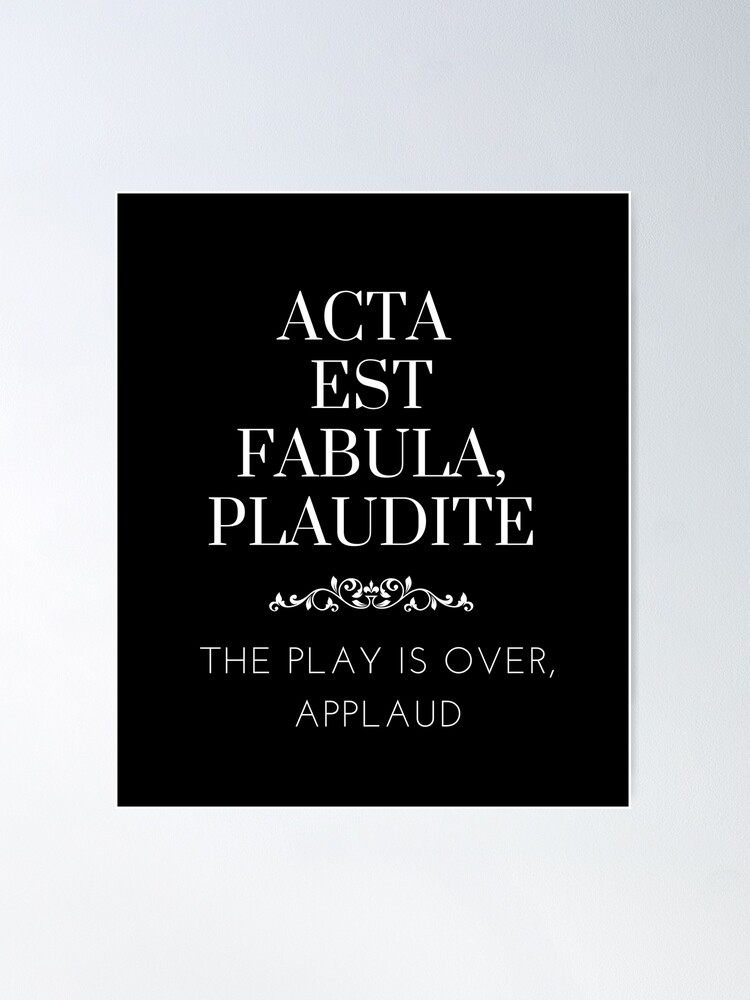This is a vertically aligned, rectangular poster with a solid black background and light gray border. The poster features a motivational message in white, all-caps lettering, centered along four lines: "ACTA EST FABULA, PLAUDITE." Below this, a decorative, swirly design resembling a woodcut pattern serves as a divider between the upper and lower sections of text. The lower section, in a thinner sans-serif font, reads: "THE PLAY IS OVER, APPLAUD." The striking contrast between the bold, serif font of the Latin phrase and the simplistic sans-serif font of the English translation adds to the visual appeal of the poster, making it both eye-catching and thought-provoking.